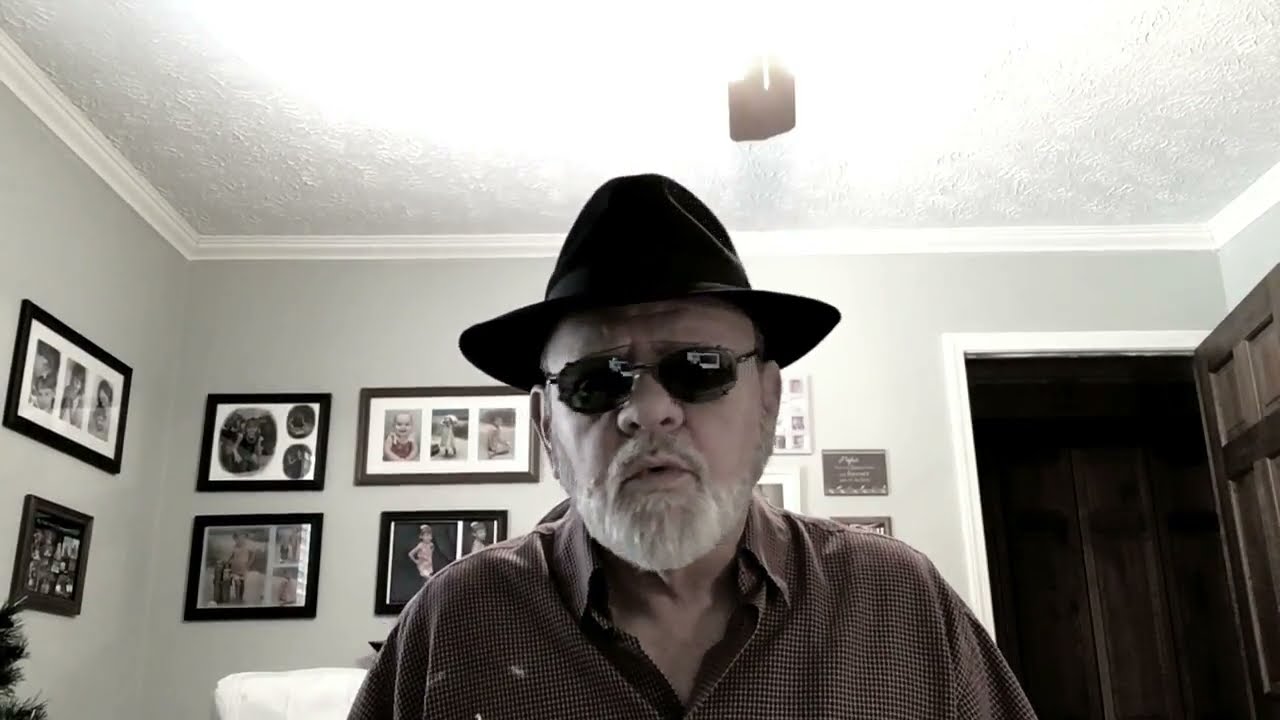This image captures an older gentleman with a white beard and mustache, donning sunglasses and a leather hat, wearing a brown shirt slightly unbuttoned at the collar. He is positioned at the center of the photo, looking directly at the camera. The scene is set indoors, likely within a living space or family room that is bathed in a brownish-cream monochrome tone, akin to a subdued sepia effect. The room features white walls adorned with numerous family photos, which seem to include pictures of children and grandchildren, creating a warm, familial atmosphere. An ornate ceiling with the light on adds an element of elegance to the room. To the gentleman's right, there is an open doorway that leads into the space, and just over his right shoulder, a plaque is visible, hinting at an achievement or award. The overall composition and elements suggest a deeply personal and intimate setting, capturing a moment in the life of the gentleman amidst his family's memorabilia.